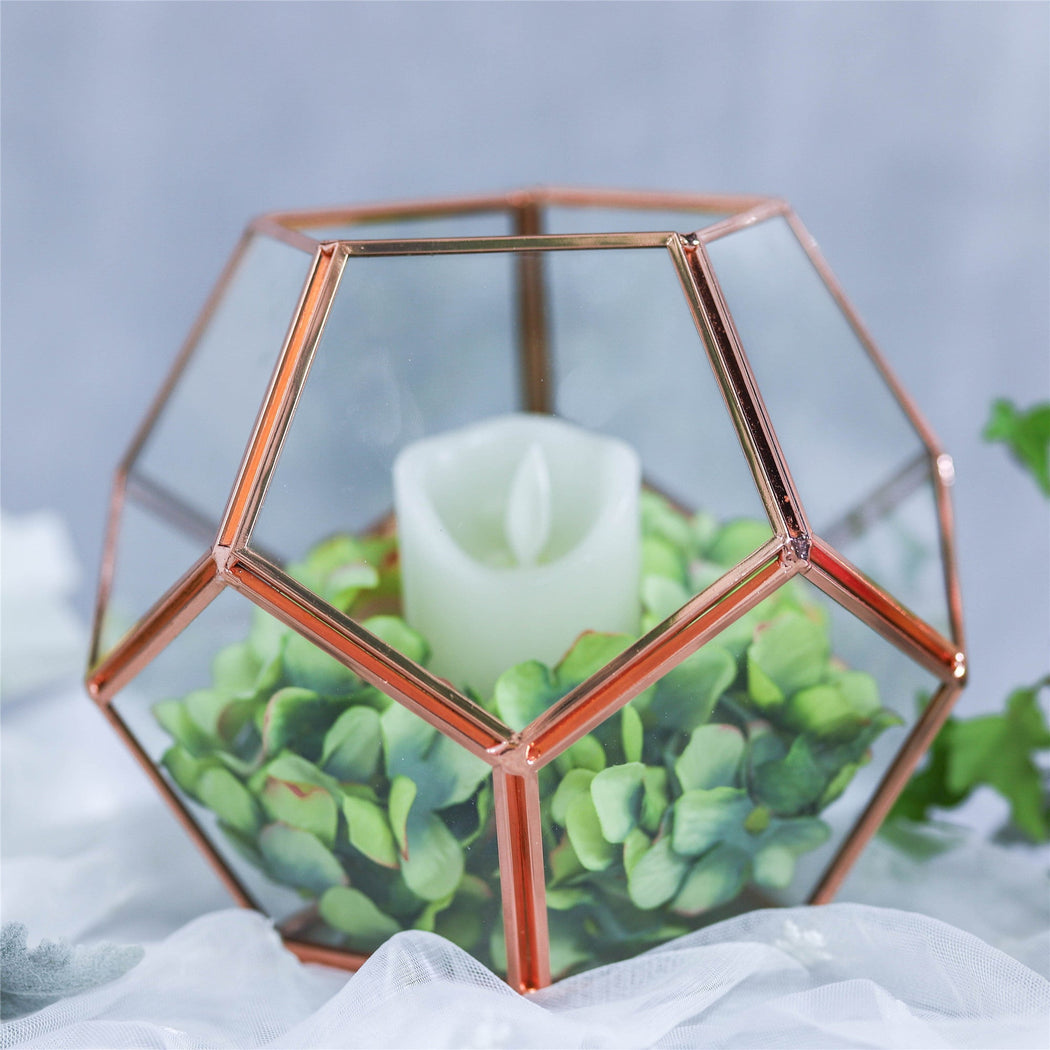A beautifully crafted geodesic candle holder made from glass and copper is captured in this image. The geometric structure features an open top, revealing a white imitation candle nestled within. Surrounding the candle are lifelike artificial leaves, adding a touch of nature to the design. The holder itself rests on a delicate, light-colored fabric that resembles taffeta. In the background on the right, additional leaves are visible, enhancing the natural theme of the composition.